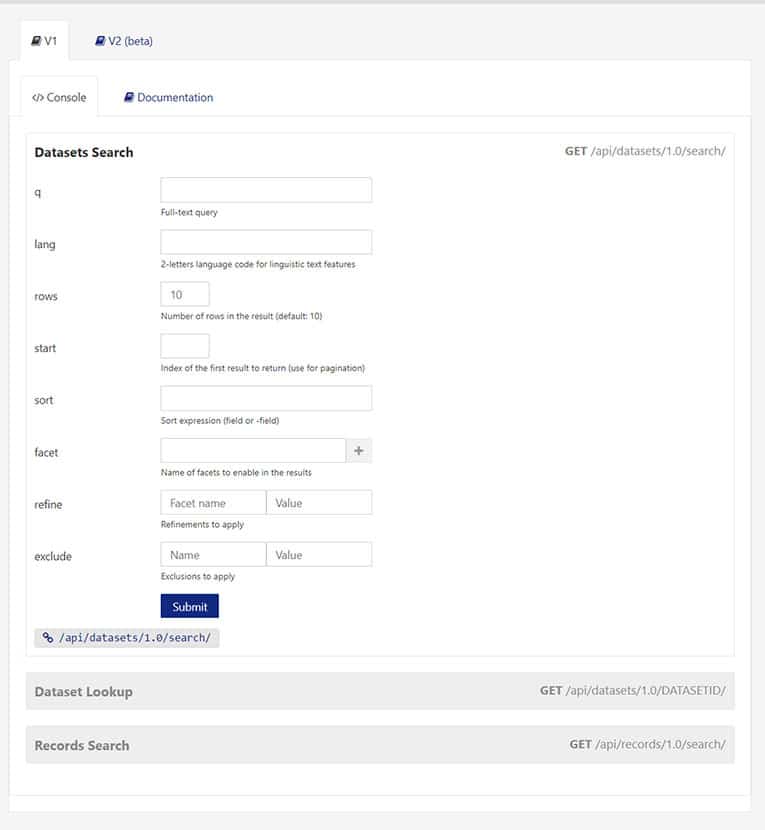Here, we have a detailed screenshot featuring a white background framed by a light gray border. At the very top, there is a series of tabs—'B1,' which is currently active, and next to it, 'B2,' which is in a lighter shade indicating it is inactive. Below this, there are two more tabs, with the 'Console' tab open and 'Documentation' tab closed.

Directly underneath the tabs, a square section with a light gray border contains the heading "Dataset Search." On the left side of this section, there is a list of terms or items (unreadable in the screenshot), each accompanied by an adjacent white input box intended for user text entry. Below each input box, there are small black letters, likely labeling or providing descriptions for each field.

At the very bottom of this section, there is a prominent blue 'Submit' button. Next to it, there is a gray button displaying a copy symbol, presumably for copying information or data.

Further down, two elongated gray bars span the width of the screenshot. The top bar is labeled "Dataset Lookup," while the bottom bar bears the label "Record Search." To the right of these bars, there is text indicating an endpoint or a URL path reading "GET /" followed by what seems to be a web address for accessing these functions.